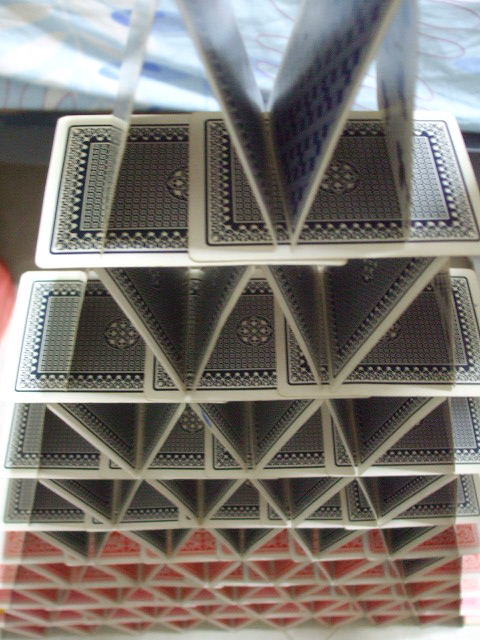This overhead photograph captures an intricate work of art constructed by meticulously stacking playing cards into a pyramid formation. The playing cards are arranged in a precise grid pattern, beginning with a broad base. At the bottom, pairs of cards are leaned against each other to form a row of triangular structures, akin to a series of interlocking grids. Each ascending layer of the pyramid narrows as the triangular formations taper towards the apex. Horizontal cards are carefully laid flat between each layer, serving both as a stabilizing platform and a support for the subsequent rows of triangles.

The pyramid culminates at the top with two visible triangular structures, flanked by two horizontal cards. The entire structure exudes a sense of precise balance and delicate craftsmanship. The cards themselves are predominantly gray and black, with the exception of a partial glimpse of a club suit on the topmost card. The background reveals a white surface upon which the pyramid rests, with hints of a white fabric visible at the upper edge of the image. This artistic photograph showcases not just the fragility of the cards, but the precision and skill involved in their careful arrangement.